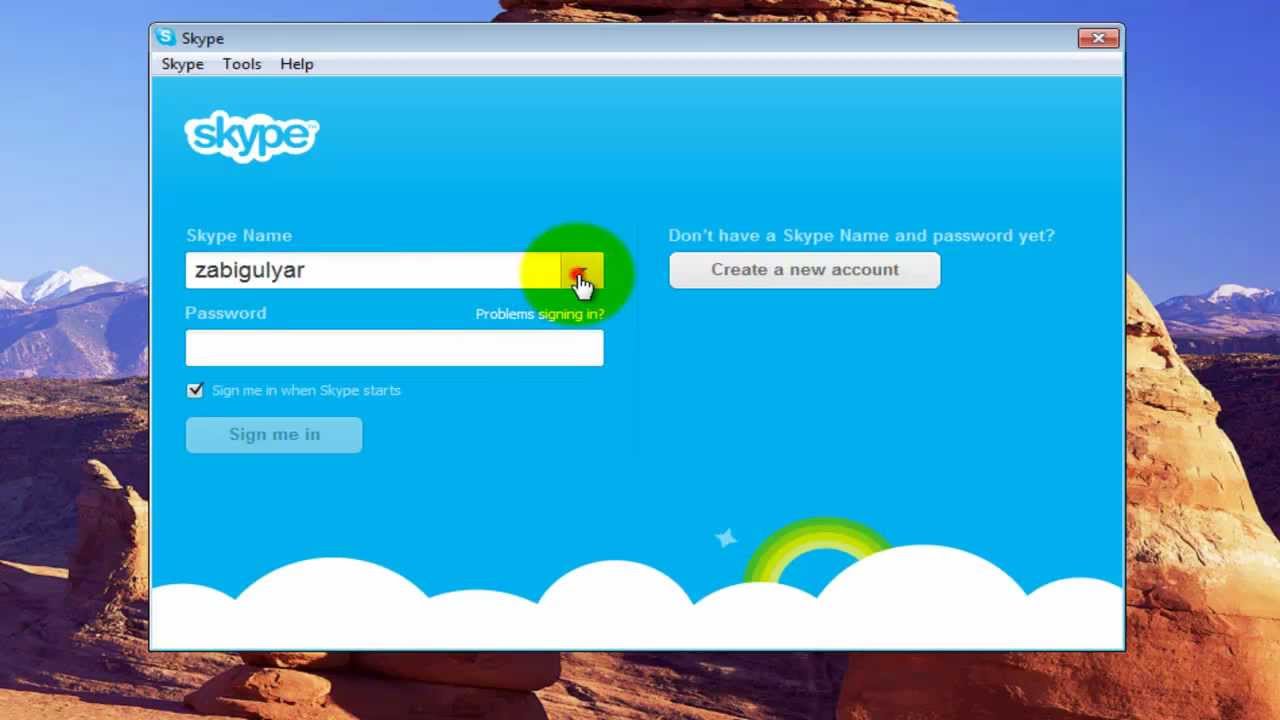The image depicts a computer screen with the Skype application prominently displayed over a mountain landscape background. The background features majestic mountains flanking the sides with a visible foreground, framing a clear, serene sky. However, the scenic view is largely obscured by the Skype interface overlay.

In the upper left corner of the Skype window, the Skype logo is visible alongside the word "Skype." Oppositely, in the upper right corner, there's a red box with a white "X" indicating the close button. Just below, the application menu includes tabs labeled "Skype," "Tools," and "Help."

The central part of the interface displays the Skype logo again, followed by the label "Skype Name." Next to this is a text box containing the username "Zabigular," with the cursor placed at the end of the name. Below this textbox is a prompt asking, "Don't have a Skype name and password yet?" which is followed by a gray button reading "Create a new account."

Continuing downward, the label "Password" is seen, accompanied by a text box where the user is expected to enter their password, though it is currently blank. Below the password field, there’s a checkbox option labeled "Sign me in when Skype starts." Further down, a lighter blue button that reads "Sign me in" is prominently displayed.

Adding a touch of whimsy to the utility-heavy display, the background also includes an image of numerous clouds, and among them, a rainbow in different shades of green can be seen arcing elegantly above the cloudy expanse.